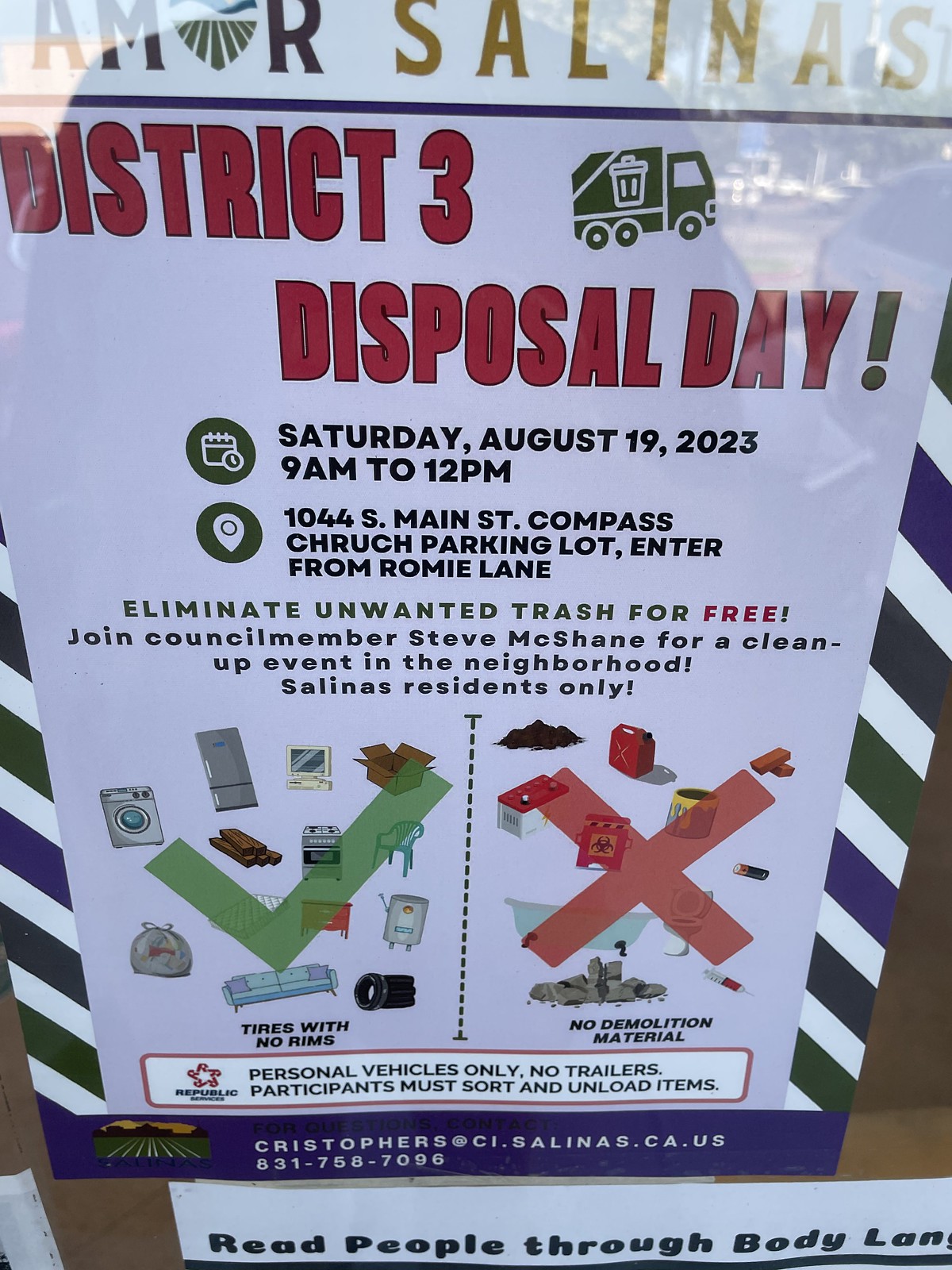The image showcases a detailed poster promoting an environmental clean-up event titled "Amor, Salinas". The poster is predominantly white, bordered with green and blue stripes. At the top, in large letters, it reads “Amor Salinas” with a stylized 'O' featuring a heart symbol. Below this, in red font, it states “District 3 Disposal Day” alongside a green exclamation point. A graphic of a green garbage truck with a garbage can is also present.

The event details are clearly laid out with a calendar icon stating, “Saturday, August 19, 2023, 9 AM to 12 PM”, and the address “1044 Main Street, Compass Church parking lot, enter from Romy Lane.” The poster encourages residents to “Eliminate unwanted trash for free” and invites them to “Join Councilmember Steve McShane for a clean-up event in the neighborhood.”

In the middle of the poster, acceptable items to bring are listed with illustrations of a washing machine, refrigerator, stove, couch, cardboard box, computer, and tires (noting “tires with no rims”), all marked with a green checkmark. Unacceptable items include a picture of a pile of dirt, a gasoline can, a biohazard sign, a paint can, a battery, a toilet, a bathtub, a needle, and demolition materials, each marked with a red X.

At the bottom, it emphasizes “Salinas residents only,” and notes “Personal vehicles only, no trailers,” along with the instruction that “Participants must sort and unload items.” Additional contact information provided includes “Christopher’s at ci.salinas.ca.us” and the phone number “831-758-7096.” The poster also features the phrase “Read people through body and lung” towards the bottom.